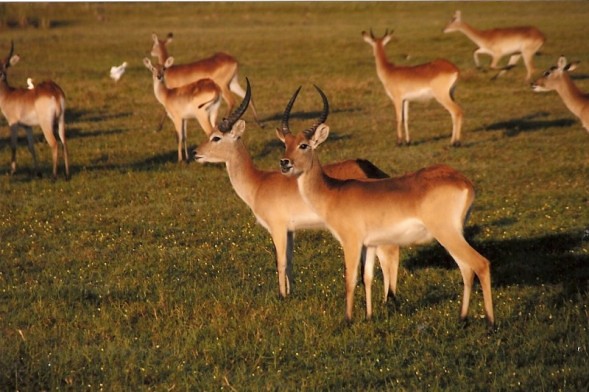A serene photograph captures a grassy meadow with green and slightly brown-tinted grass, accented by tiny yellow flowers near the center. The scene is dominated by a group of seven antelope, with just the head of an eighth visible. To the right and just above the center, a dark brown antelope with one prominent long black horn intrudes into the frame. This antelope has white at the top of its back legs, which turn black towards the bottom. Behind and slightly to the right stands another antelope, its tail swinging around its front. This hornless creature with erect ears is brown and light brown. Following it is another light and dark-brown antelope, facing away, revealing small black horns. Upwards and further back, an antelope runs from right to left, head forward, without antlers, displaying a light brown coat. To the right, another head peeks in, identifiable only by its ears and neck, both light brown. Closer to the foreground and central in the image, two antelopes stand together. The one on the left, partially obscured, has a single black horn and a dark brown head. In front is the largest gazelle, chest facing left and tail right, with two long black horns and a mix of light brown and dark brown fur. The backdrop suggests a distant grassy or foliage area in the upper left, and interestingly, a white figure resembling a chicken stands out, adding a unique detail to this rich, natural tableau.